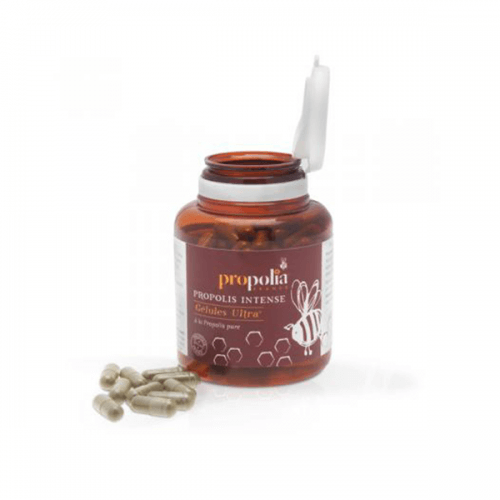The image features a clear pill bottle with a dark red sheen, topped with an open white plastic cap that is still attached to its neck. The bottle's label prominently displays the text "Propolia," followed by "Propolis Intense" and "Cellulous Ultra," though the smaller text beneath this is difficult to discern. At the bottom right corner of the label, a cartoon bee is illustrated, accompanied by honeycomb hexagon patterns to its left. The bottle itself is situated on a white background, enhancing the visibility of its contents. Approximately eight light bronze-colored capsules are scattered around the base of the bottle. These pills are cylindrical with rounded ends and suggest a natural supplement or probiotic composition. The overall aesthetic of the label is burgundy with white imagery and text, with some yellow elements in the typography.